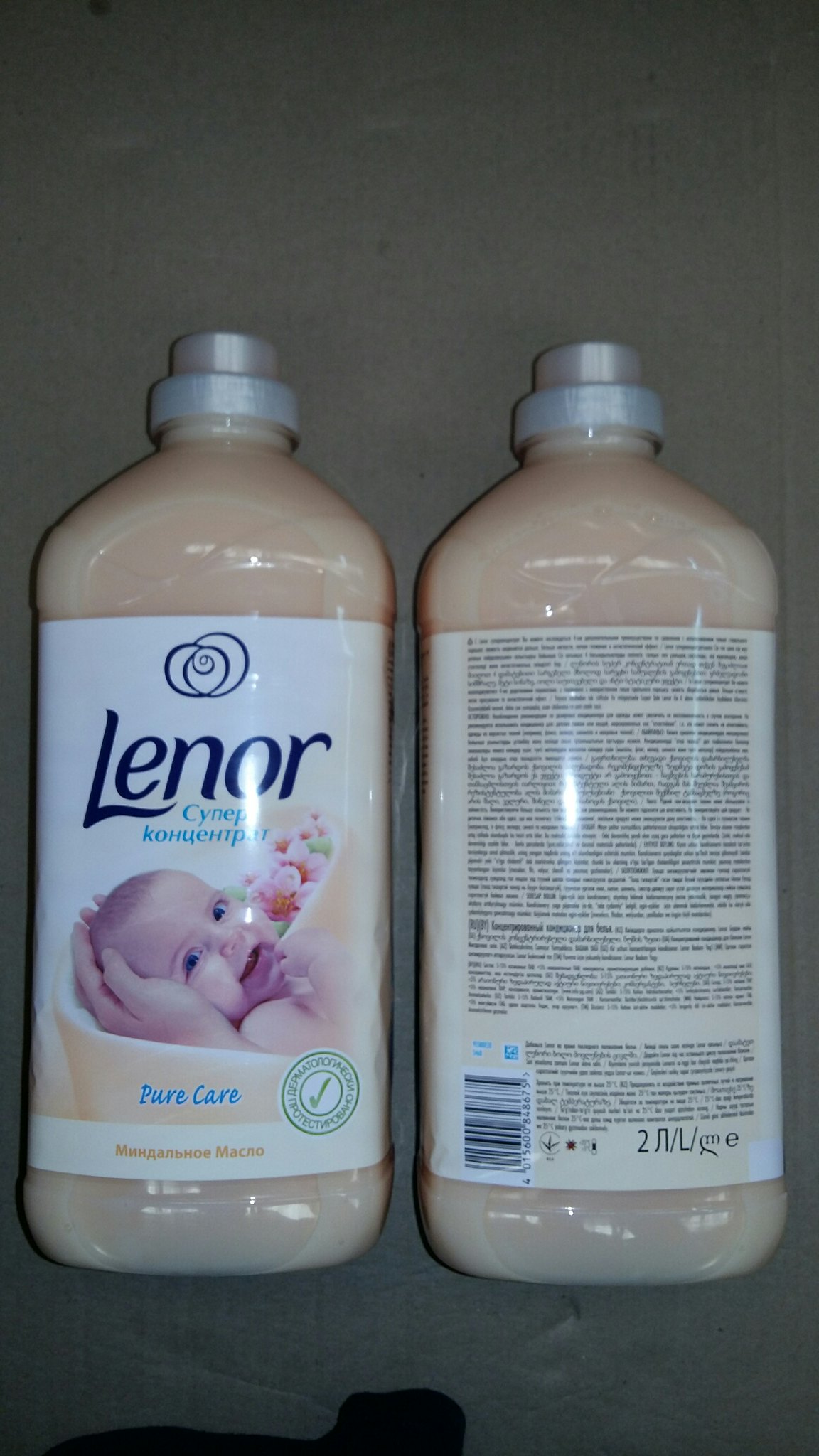Here is a comprehensive and detailed caption for the image:

"In this image, there are two bottles of Linor fabric softener placed side by side. The bottle on the left is shown from the front, while the bottle on the right displays the backside. The product, potentially of Greek or Russian origin based on the non-English text, prominently features the Linor logo along with the phrase 'Pure Care.' The bottles are transparent, encased in a plastic wrapper that includes an image of a baby's head cradled in a mother's hands, highlighting that the product is hypoallergenic and suitable for infants. The back of the right-hand bottle is densely packed with text, characteristic of many household and medical products, making it challenging to read the finer details."